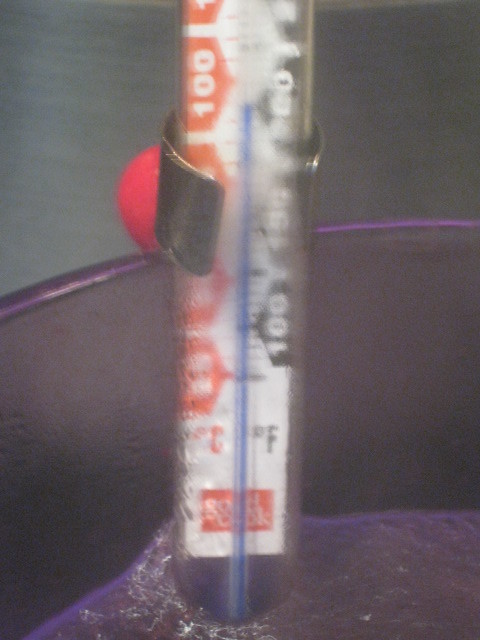The image showcases a thermometer designed for measuring liquid temperatures. The thermometer is immersed in a purple bowl filled with a clear liquid, which appears purplish due to the reflective color of the bowl. The thermometer itself is transparent, featuring red numbers on the left and black numbers on the right. The temperature-measuring liquid inside the thermometer is blue, indicating a temperature close to 100 degrees. A metal clamp secures the thermometer to the bowl, with a pink ball attached behind the clamp, possibly serving as a stabilizing mechanism. The background is pitch black, providing a stark contrast to the vibrant foreground elements. Condensation is visible at the bottom of the thermometer, further emphasizing the presence of liquid.